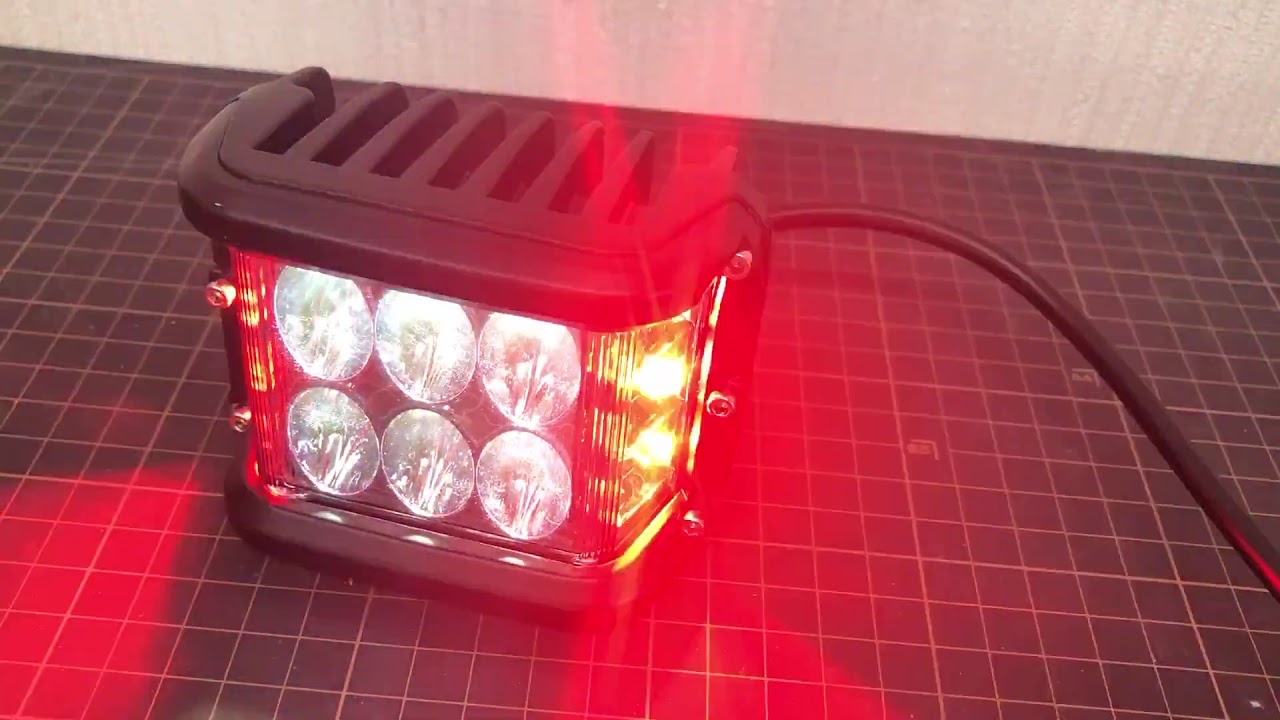The image features a compact and durable black plastic housing of a vehicle light assembly, typically found on off-road vehicles. The central component comprises six bright white lamps at the front, complemented by red and orange side lights. This light assembly, which may be undergoing testing or assembly, is placed on a dark grid-patterned table, resembling a cutting mat. Connected to the housing is a thick cable extending to the right, likely for powering the unit. The background consists of a plain white wall, highlighting the light assembly, with additional visible details including metal screws fastening the housing and thin vents at the top to dissipate heat. The scene's color palette includes shades of red, orange, yellow, black, gray, and a light tan, with the striking combination of the light and housing drawing primary attention in the image.